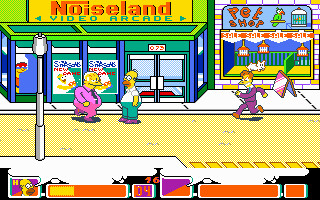In this highly colorful and pixelated screenshot reminiscent of 90s or early 2000s video games, we see a vibrant scene from a retro-looking Simpsons side-scrolling beat-em-up game. The setting is a city street, where Homer Simpson, in his signature white shirt and blue pants, stands prominently in the center of the screen. He is positioned outside a yellow and green storefront labeled "Noiseland Video Arcade," with an adjacent pet shop featuring a bird logo and a caged bird visible. 

Homer appears to be engaged in conversation with a large, portly man dressed in a purple suit with white hair and a tie, located to his left. Simultaneously, another character—a man in a purple suit with orange hair bearing an angry expression—is seen running towards Homer from the right edge of the screen. The bottom of the screen displays Homer's health bar and another unused health bar, suggesting the presence of a yet-to-be-activated Player 2. The image's overall color palette includes striking yellows, oranges, greens, and blues, evoking the cartoonish video game style of the late 90s and early 2000s.